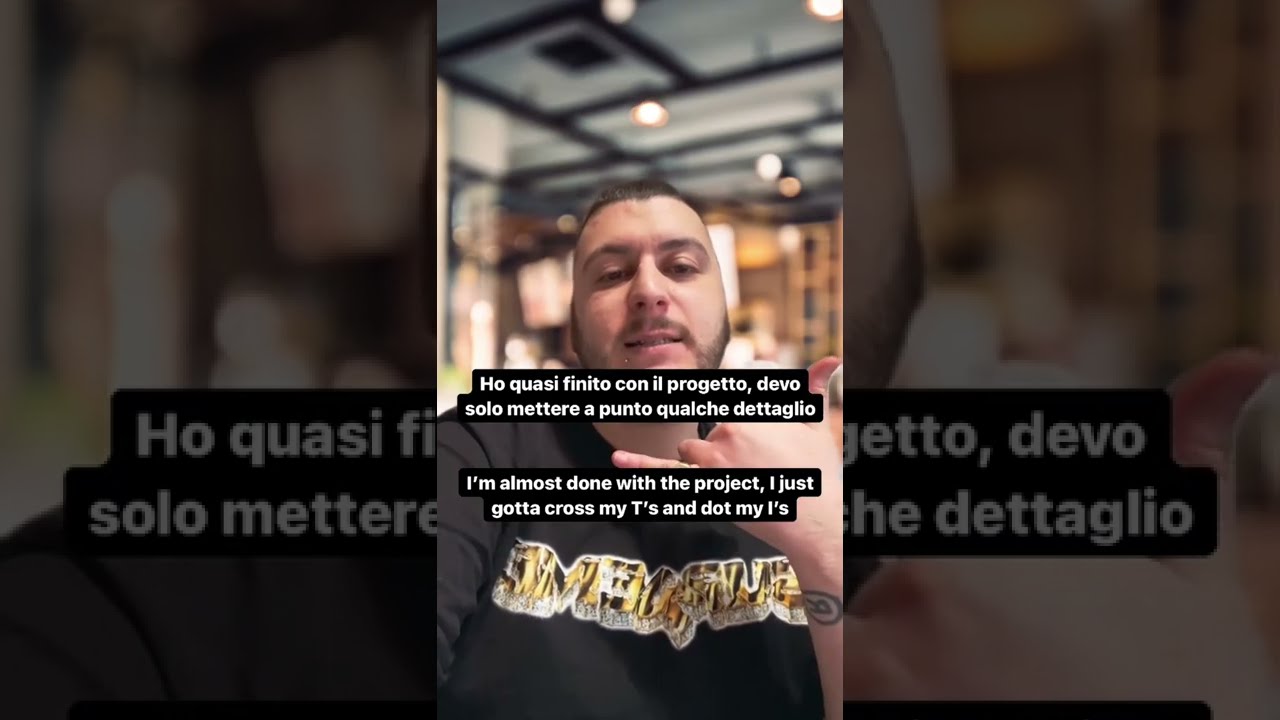The image features a man, potentially an adult male of Caucasian or Middle Eastern descent, who is taking a selfie or possibly a video screenshot. He has a neatly trimmed small brown beard and very short brown hair. He is wearing a black t-shirt with a tiger stripe logo and some yellow lettering across the center, though the exact text is unclear. He is making a "shaka" sign with his hand, extending his thumb and pinky finger, and is staring directly at the camera with a light complexion enhanced by shining light. There is an indication of a tattoo on his left wrist. The background appears to be a public setting like a coffee shop or office, featuring blurred lights and cabinets, giving it a somewhat celebratory atmosphere.

Overlaying the image are white subtitles with a black background. The top text is in Italian, reading "Ho quasi finito con il progetto, devo solo mettere a punto qualche dettaglio," which translates to "I'm almost done with the project, I just gotta cross my T's and dot my I's" in English. The image also has a decorative border on the left and right sides, created by enlarging and darkening elements of the main image.